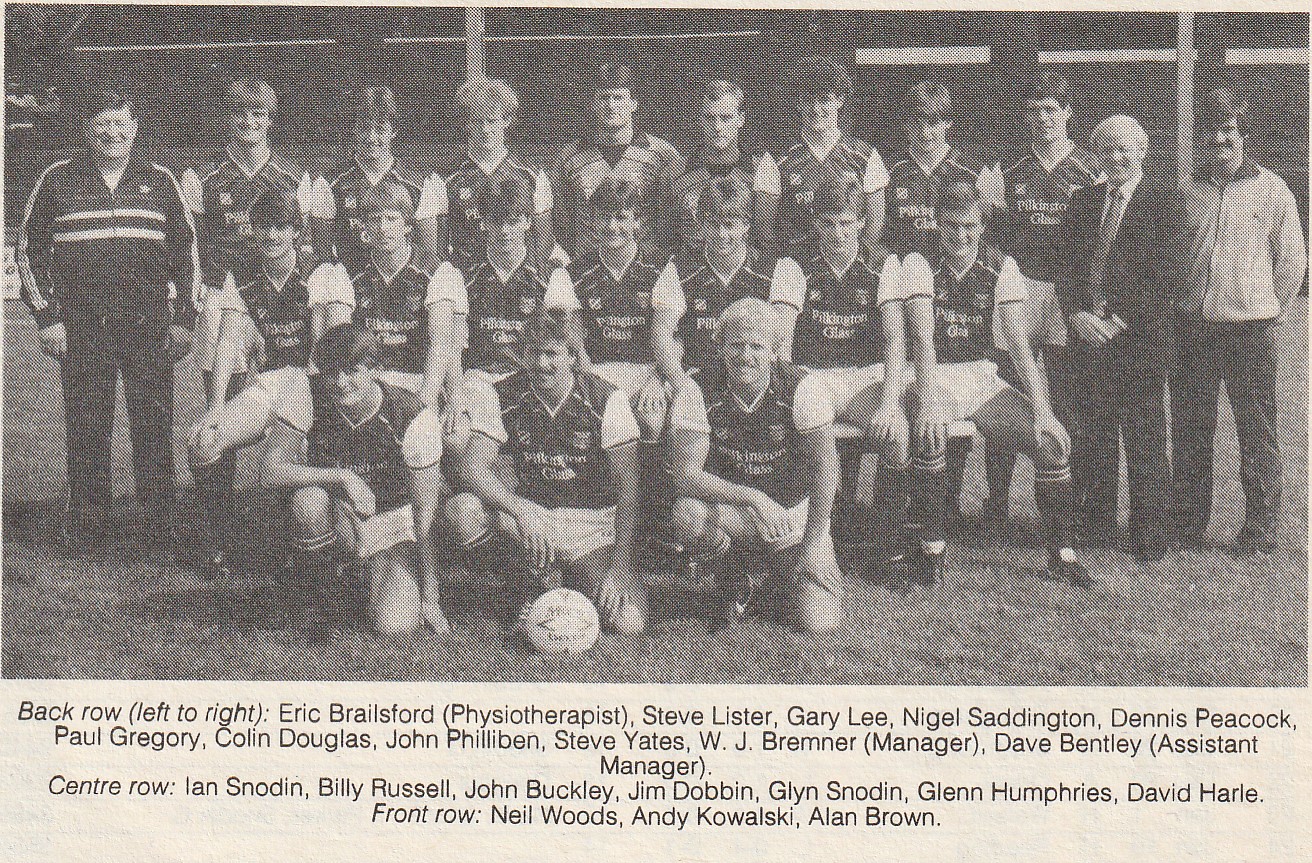The black and white photograph, likely an excerpt from a newspaper or magazine, showcases an old-fashioned soccer team arranged in three distinct rows. The top part of the image prominently features this photograph, capturing the team members in various poses. The team, consisting of older men in darker colored jerseys with white sleeves and white shorts, includes different roles identified by their attire. In the first row, three players are kneeling; the second row, consisting of seven players, are sitting on a bench; and the last row, which has eight standing players, completes the formation. 

To the left stands an older man in a striped tracksuit jacket paired with black pants, identified as a physiotherapist, while on the right side, one man in a business suit and tie stands next to another in a checkered jacket and black pants. Details such as the presence of mustaches suggest a specific era.

Beneath the photograph, on what appears to be a beige piece of paper, the caption lists the team's members' names in small, italicized black font. It starts with the "back row, left to right", mentioning Eric Brailsford, the physiotherapist, followed by other names like Steve Lister and Gary Lee. It proceeds to name people in the center row and front row, also identifying key figures such as the manager, W.J. Bremer, and the assistant manager, Dave Bentley.